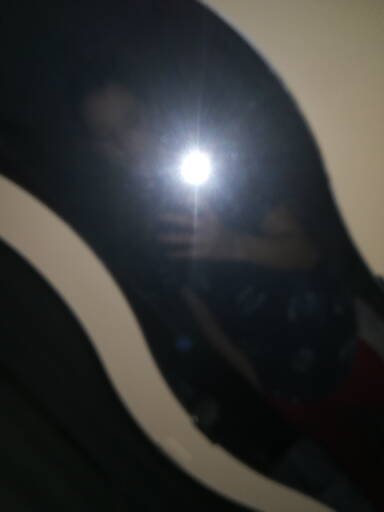In this image, a person is taking a selfie in front of a mirror. The individual, who appears to be male and of slim build, is holding a smartphone vertically, with their hand visible at the bottom of the device. The flash from the phone is incredibly bright and prominent, casting a stark illumination over the scene. The photograph is slightly tilted, giving it a dynamic and somewhat casual feel. Due to the darkness of the room, details about the person's features and hair are difficult to discern. The powerful flash, however, accentuates the contours of their face and hand, suggesting that they are possibly posing for a portrait-style photo.